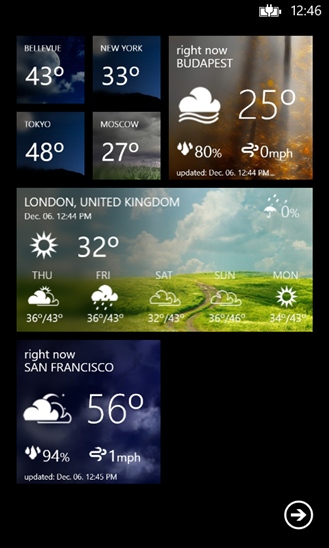The image features a digital weather display on a screen with a black background. At the top left corner, there are four small squares representing different locations and their respective temperatures: Bellevue at 43°F, New York at 33°F, Tokyo at 48°F, and Moscow at 27°F. To the right, the screen shows Budapest at 25°F with an 80% chance of precipitation and no wind. 

Centered below is a rectangular section displaying weather information for London, United Kingdom: the current date is December 6th, 12:44 PM, with a temperature of 32°F and sunny conditions. The forecast spans from Thursday through Monday. 

Below the London section, in a dark blue square, is the weather for San Francisco, showing 56°F and cloudy conditions with a 94% chance of precipitation and wind speeds of 1 mph.

The top of the screen also shows a full battery icon on the left and the current time, 12:46, on the right. At the bottom right of the screen, there is a white circle with a white arrow pointing to the right.